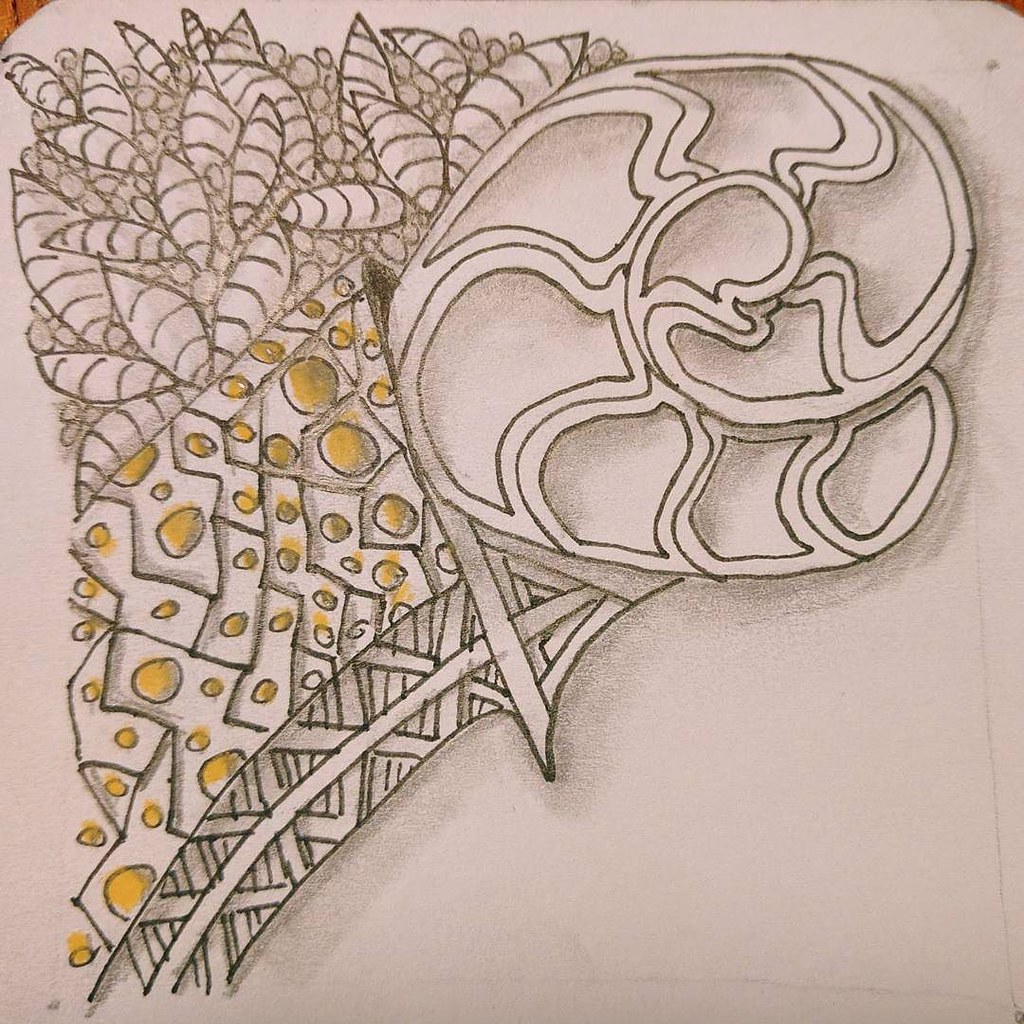This is a photograph of an abstract, hand-drawn piece of art on white paper, characterized by intricate details and a combination of colored pencil and shading techniques. The central feature of the drawing is a cutaway of a Nautilus shell, which seamlessly transitions into a large, circular, floral or fan blade-like design with a flowing, spiraling pattern. This key element is surrounded by numerous randomly positioned geometric shapes, each containing small yellow-colored circles. Extending from the Nautilus and geometric shapes is an arrow-like structure, designed with a cross-hatch pattern resembling wooden girders. Above this section, a collection of abstract, black and white leafy structures or crescent-shaped forms adds complexity to the composition. The drawing also includes several smudged areas and visible paper wrinkles, giving it a raw, unfinished aesthetic. The overall image combines elements of geometry, organic forms, and abstract shapes, unified by a cohesive interplay of black, white, and yellow.